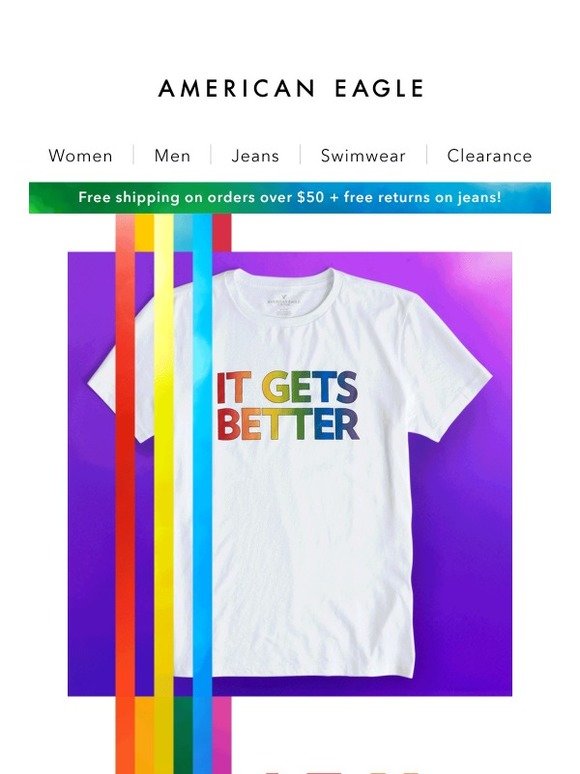This screenshot captures an American Eagle advertisement, likely sourced from a website, set against a predominantly white background. At the top, prominently displayed in bold black letters, is the brand name "American Eagle." Directly beneath this, five black category labels—"Women," "Men," "Jeans," "Swimwear," and "Clearance"—are separated by thin vertical gray lines for clear navigation.

A striking horizontal bar in shades of green transitioning to blue spans the width below the categories. Bold white text within this bar announces, "Free shipping on orders over $50 plus free returns on jeans," making a compelling offer to potential customers.

The area below features a vivid purple background, centering attention on a white t-shirt adorned with colorful, multicolored letters forming the phrase "It Gets Better." This positive message is emboldened by the vibrant hues of the letters: the "I" in red, "T" in red, "G" in yellow with a gradient to green, blue, and a deeper blue, and the rest of the letters carrying through with a mix of yellow, green, and blue shades.

Adjacent to this central image, on the left side, three vertical color bars add a dynamic and eye-catching touch, extending beyond the confines of the screenshot. These bars are colored red, yellow, and turquoise blue from left to right, contributing to the ad's overall colorful and uplifting design.

The detailed coloring of the t-shirt's slogan mirrors the energetic color scheme, incorporating reds, yellows, greens, and blues in a gradient and patterned style, enhancing the vibrant and inclusive message of the advertisement.